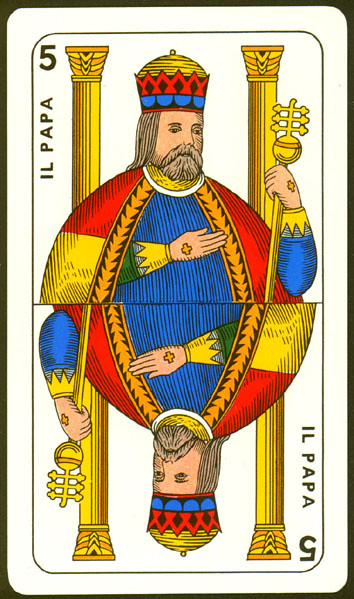Here's a more detailed and cleaned-up descriptive caption for the image:

---

This image showcases a playing card designed with a mirrored layout, creating a symmetrical appearance from top to bottom. The card itself is a long rectangle with a black border and rounded corners. Within this outer border lies another white, rounded rectangle. Encased inside this frame is yet another rounded rectangle containing the central illustration and text.

The card displays a regal figure identified as "Il Papa," or The Pope, dressed in a rich yellow and red cloak. The right side of the cloak, near his right arm, features intricate black details adorned with orange, downward-pointing arrowheads that interlock. This figure also bears small yellow cross tattoos on the wrists of both hands.

He is clad in a blue shirt beneath the cloak, with green sleeves ending in jagged yellow cuffs. He holds a commanding staff topped with a yellow orb, outlined in orange, and decorated with three prongs extending from it.

Behind The Pope stand two substantial pillars, colored yellow and orange, enhancing the stature of the central character. The card's denomination, represented by the number 5, is positioned in the top left corner and again in the bottom right corner, but inverted. The card title "Il Papa" appears along the left edge at the top and is mirrored along the right edge at the bottom.

Thus, the design creates a mirrored effect where the top half of the card is exactly duplicated in an inverted form at the bottom half.

---

This cleaned-up version aims to provide a clear and comprehensive description while maintaining the intricate details of the card's design.